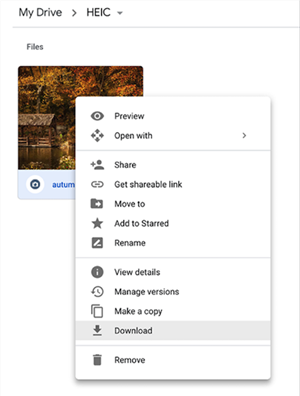A blurry screenshot likely taken from a smartphone depicts a mixture of graphic elements and text. The background of the image is a blend of shades of brown and orange, suggesting an autumn theme. Embedded in the background is a faint icon, indistinct in its form, and the word "autumn" is partially visible.

The foreground is dominated by a partially translucent overlay containing text and menu options. At the top of the screen, the text reads "This is my drive," followed by an arrow indicating a dropdown menu. To the right, the text "H-E-I-C" appears, also accompanied by an arrow, suggesting the presence of another menu.

An open dropdown menu below these headings offers a variety of options: "Preview," "Open with" (with a subsequent arrow for further selections), "Share," "Get shareable link," "Move to," "Add to start," "Rename," "Details," "Manage versions," "Make a copy," "Download," and "Remove." The word "files" appears above the blurry image, indicating the context of file management. The overall image presents a layered, visually complex screenshot of a digital file management interface on a smartphone.